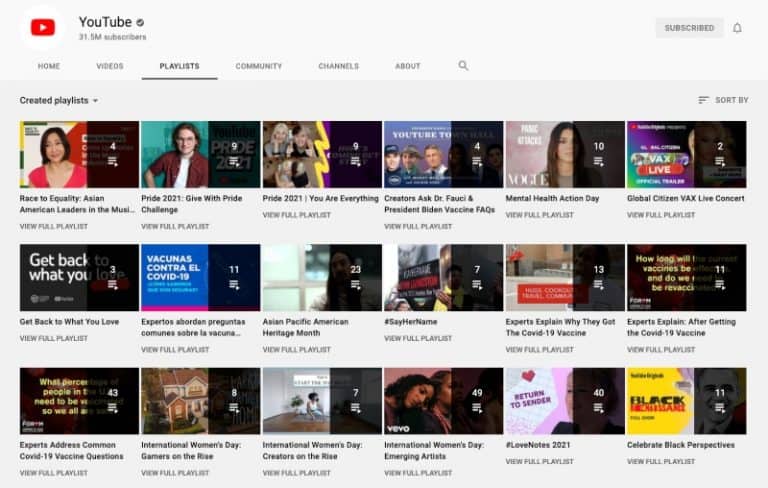Here is your revised descriptive caption:

---

This image is a detailed screenshot of a YouTube user's account interface displayed on a predominantly white background. In the upper left-hand corner, the iconic red YouTube play button is visible, accompanied by the word "YouTube" in black lettering next to the text "31.5 million subscribers." 

Below this, on the left side of the screen, is a labeled menu bar featuring options such as Home, Videos, and Playlists, with the Playlists tab highlighted by an underscored black line. Additional tabs include Community, Channels, About, and a search icon represented by a magnifying glass.

In the upper-right corner, the interface displays a "Subscribed" button alongside a gray notification bell icon. 

The main content area is an off-white gray section organized into three rows and six columns of video thumbnails. At the top of this section, the label "Created Playlists" is prominently displayed. The thumbnails showcase various video topics, with titles such as "Race to Equality," "Asian American Leaders in Music," "Pride 2021," and "Give with Pride Challenge" in the first row. The second row includes videos like "Get Back into What You Love" and "Asian Pacific American Heritage Month." The final row starts with "Experts Address Common COVID-19 Vaccine Questions" and concludes with "Celebrate Black Perspective" on the far right.

This image provides an insightful glimpse into the diverse range of playlists and video themes featured on a YouTube channel boasting a substantial subscriber base.